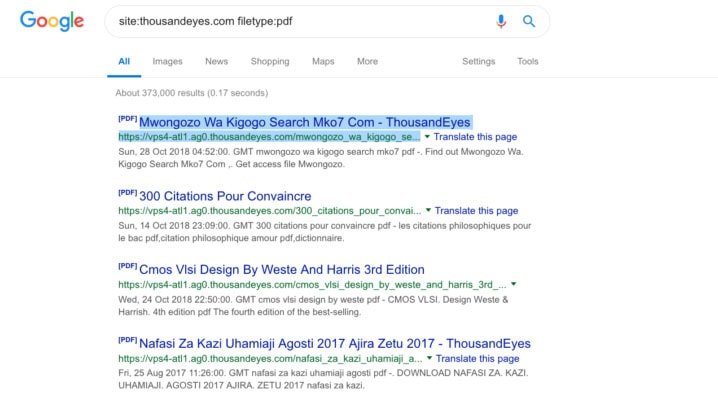This image captures a Google search results page, prominently showcasing the Google logo in the upper left corner. The logo features a capital blue "G" followed by lowercase letters: a red "o," a yellow "o," a blue "g," a green "l," and a red "e." To the right of the logo, there's a search bar containing text related to "ThousandEyes.com" and a PDF file. Below the search bar are various navigation tabs for "All," "Images," "News," "Shopping," "Maps," and "More," with "Settings" and "Tools" options on the far right. The search results indicate approximately 373,000 results were found in 0.1 seconds. The first few results displayed are PDF files, with the first result highlighted in blue.